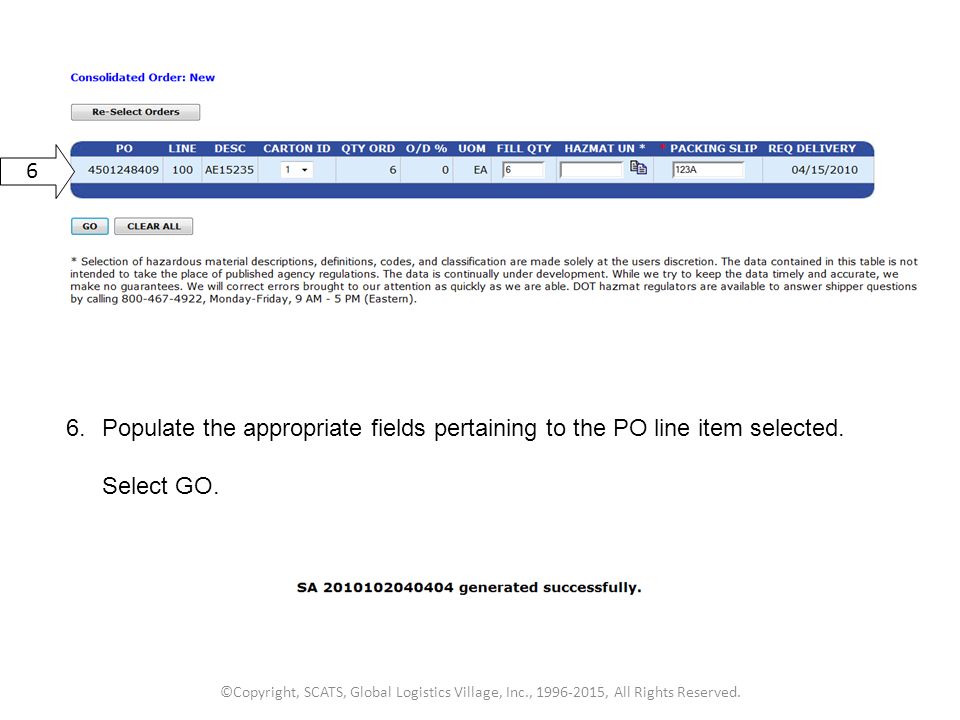The image is a screenshot of a section of an order form. At the top of the image, the title "Consolidated Order, New" is displayed prominently in purple text. Adjacent to the title is a button labeled "Reselect Orders." 

Directly beneath this is a blue bar, and within this section, a white arrow labeled with the number '6' points to a Purchase Order (PO) number: 4501248409. Additional order details are listed as follows:

- **Line Number:** 100 
- **Description (DESC) Number:** AE15235 
- **Carton ID:** 1 (with an accompanying drop-down menu for further options) 
- **Quantity Ordered:** 6 
- **O/D Percent:** 0 
- **Unit of Measure (UOM):** EA 
- **Fill Quantity:** 6 
- **Hazmat UN:** (Not filled in) 
- **Packing Slip Number:** 123A 
- **Requested Delivery Date:** April 15, 2010

The overall layout provides a clear, organized summary of the specific order details, enhancing the user's ability to review or adjust the order as needed.